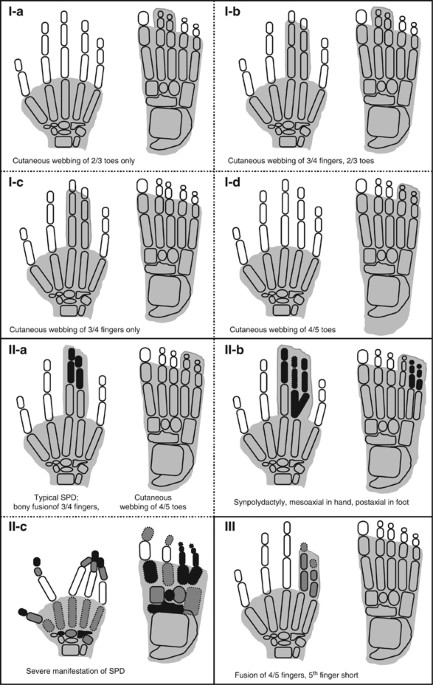The image is an eight-paneled infographic divided into two columns, each containing four panels. Each panel includes X-ray outlines of a left hand and a left foot, showing various forms of skeletal and cutaneous webbing. The panels are labeled from I-A to I-D in the first column, and from II-A to II-I in the second column, with detailed annotations:

- The first panel (I-A) describes "cutaneous webbing of 2-3 toes only," illustrating minimal toe webbing.
- The second panel (I-B) shows "cutaneous webbing of 3-4 fingers and 2-3 toes,” indicating both finger and toe webbing.
- The third panel (I-C) is labeled as "cutaneous webbing of 3-4 fingers only," focusing on finger webbing without toe involvement.
- The fourth panel (I-D) highlights "cutaneous webbing of 4-5 toes," solely depicting extensive toe webbing.
  
In the second column:

- The panel labeled II-A shows a more complex condition with "typical SPD, bony fusion of 3-4 fingers, continuous webbing of 4-5 toes."
- The panel labeled II-B describes "SYMPOLYDACTYLY: mesoaxial in hand and postaxial in foot," suggesting a specific pattern of webbing.
- The II-C panel indicates "severe manifestations of SPD," showing significant distortions in both hand and foot.
- The final panel (II-I) details "fusions of 4-5 fingers, 5th finger short," depicting substantial skeletal alterations.

Overall, the infographic illustrates various syndromic conditions related to webbed digits (syndactyly) and their severity, highlighting different patterns of webbing and skeletal fusions in hands and feet.